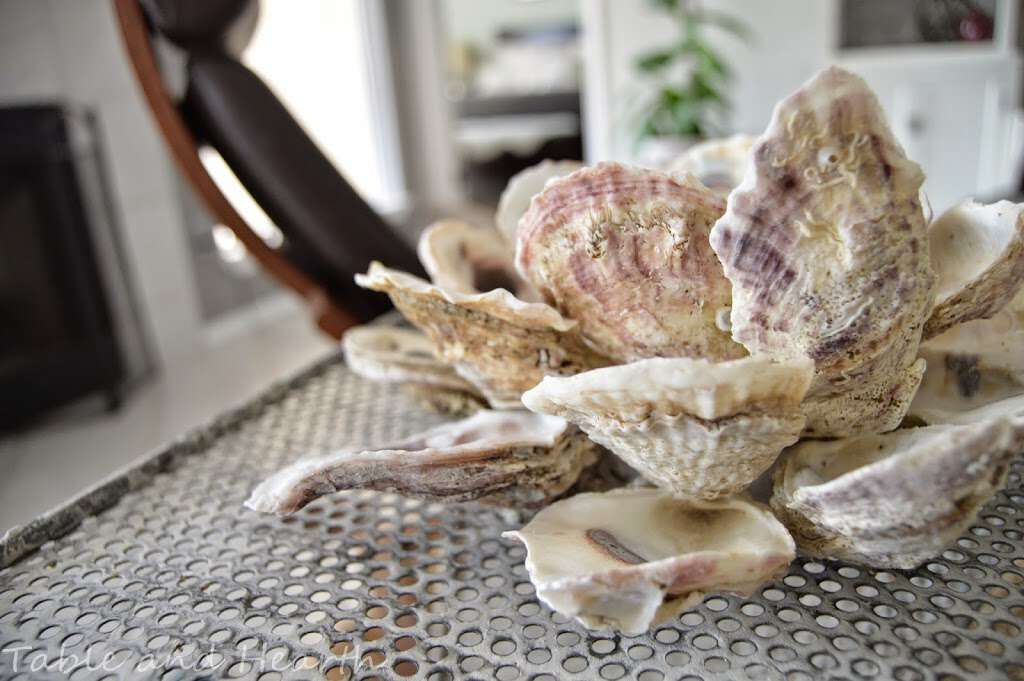In this vibrant indoor color photograph, a collection of seashells, possibly mollusks or mussels, is prominently displayed on a wire mesh rack filled with holes, designed to drain water. The shells are stacked and leaning against one another, forming a picturesque pile. They are predominantly creamy white on the inner side, while their external surfaces exhibit an array of hues including purples, browns, and pinkish reds, with some shells showing brown or dark red stripes. The overall effect is a harmonious blend of pastel and earthy tones, with the shells appearing fresh and crusty.

The background of the image, though blurry, reveals an indoor setting featuring white walls and a plant in the corner, with sunlight streaming in from a window. There is also a white cabinet visible in the top right corner and a curved, black and brown object—possibly a chair—positioned behind the rack of seashells. A bed or couch is slightly discernible in this well-lit, cozy room, adding to the homey atmosphere of the scene.